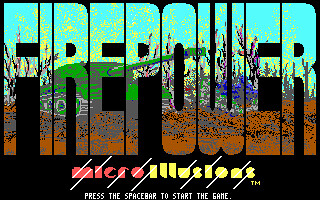Title screen for the game "Firepower," featuring a graphic drawing. The bottom banner displays the trademark "MicroIllusions" alongside the prompt "Press the Spacebar to Start the Game." The game's title, "Firepower," dominates approximately three-fourths of the page, with the letters arranged vertically from top to bottom. The background is black, providing a sharp contrast to the title lettering. Inside the title letters, an image of a tank maneuvering over rugged terrain is rendered, adding a vivid and dynamic visual element to the screen.